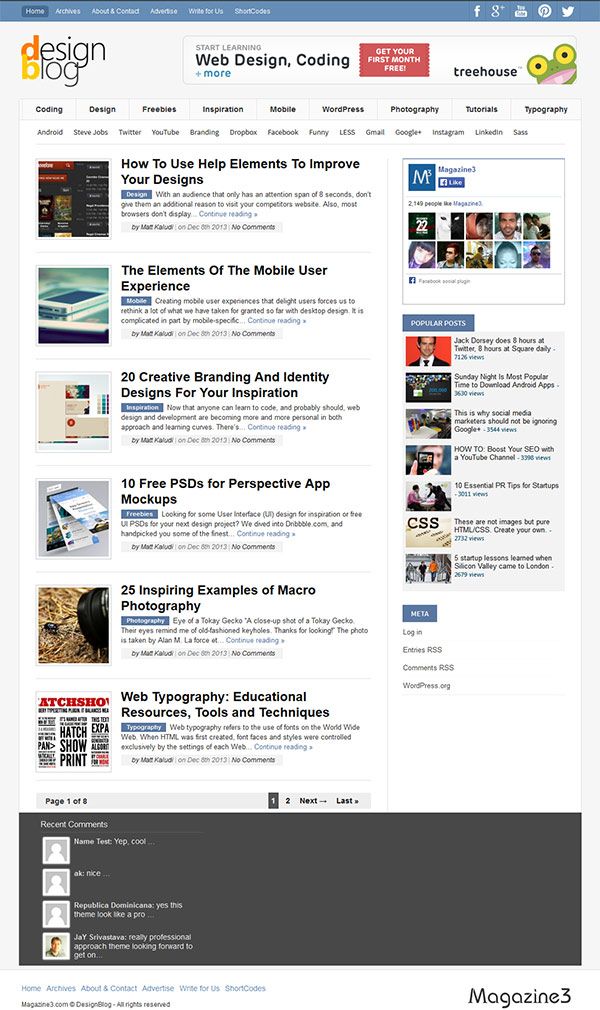At the top of the image, a long blue bar spans horizontally, featuring a lowercase "f" for Facebook on the right side, followed by a white bird icon for sharing on Twitter. Moving down to the left, the text "Design Blog" can be seen, with an orange "D" and a yellow "B." To the right of this, the words "Web Design Coding" are displayed.

Adjacent to the text is the word "Treehouse," accompanied by an image of a frog with large, circular yellow eyes and black pupils. Below this, there is a black box with the text "How to Help Elements to Improve Your Designs" next to it.

Continuing downward, an image of an iPad on a table appears with the caption "The Elements of the Mobile User Experience." Beneath this, the text "20 Creative Branding and Identity Designs for Your Inspiration" is displayed. Further down, "10 Free PSDs for Perspective App Mockups" is listed, followed by "25 Inspiring Examples of Macro Photography."

At the bottom, the text "Web Typography: Educational Resources, Tools, and Techniques" appears, and finally, a long gray square spans the bottom of the image, containing what looks like four different lines of conversation in white text.